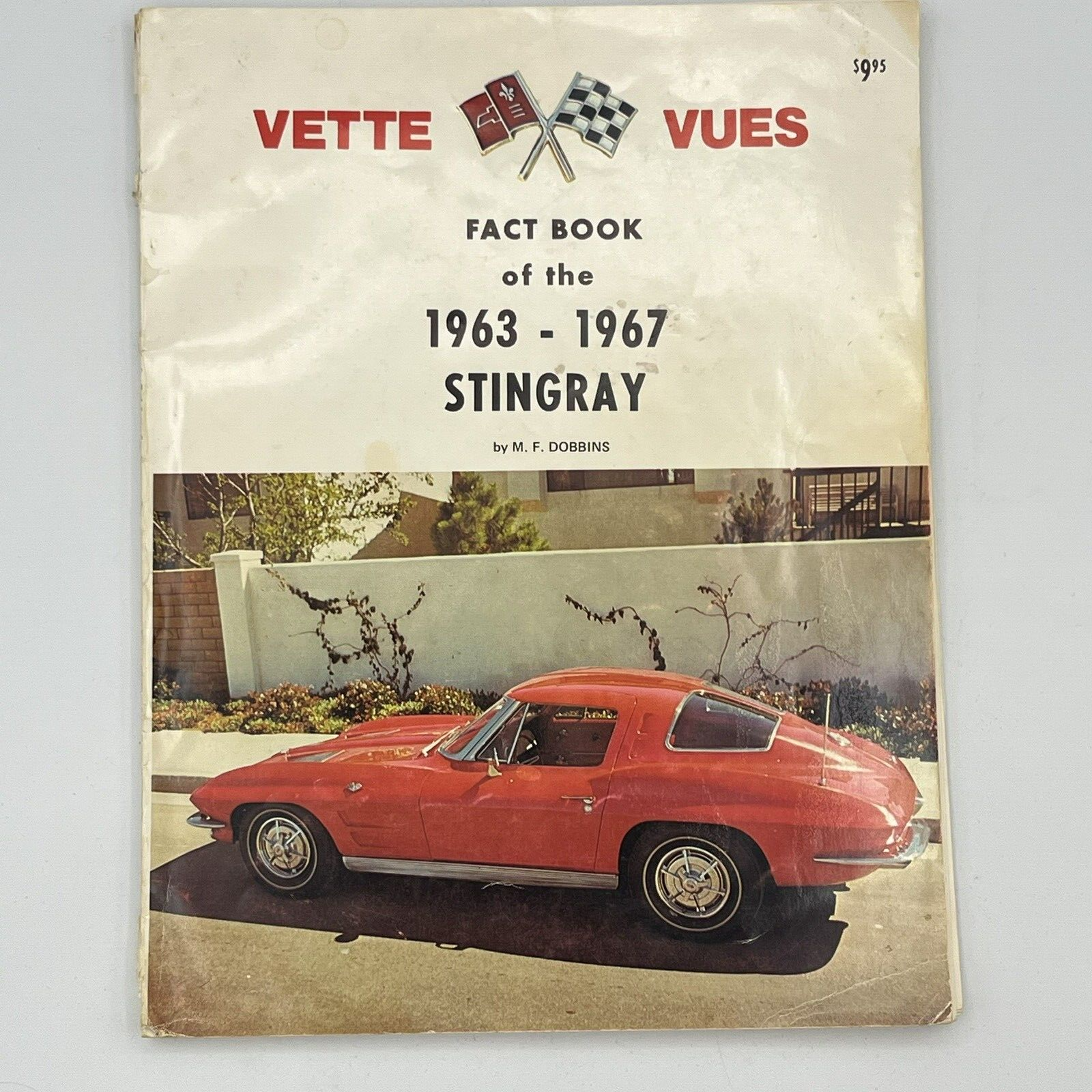The image features a vintage fact book cover for the Corvette Stingray, detailing the years 1963 to 1967. At the top of the cover, against a white background, the red text reads "Vette Vues." Centrally located between these words are two metal pin flags: a black and white checkered racing flag and a red flag bearing the Ford logo, crossed in a dynamic, motion-like design. In the top right corner, the price of the book is marked as $9.95 in black. Below this, in simple black font, the text reads "Fact Book of the 1963 to 1967 Stingray" by M.F. Dobbins. The bottom half of the cover features an image of a pristine, shiny red Stingray coupe, angled left and parked beside a slightly raised white sidewalk. The setting appears to be a residential area with an ivy-clad white wall, a brown brick post, and a building in the background, possibly an apartment complex. The scene is captured in the daytime, suggesting afternoon lighting based on the car's shadow.